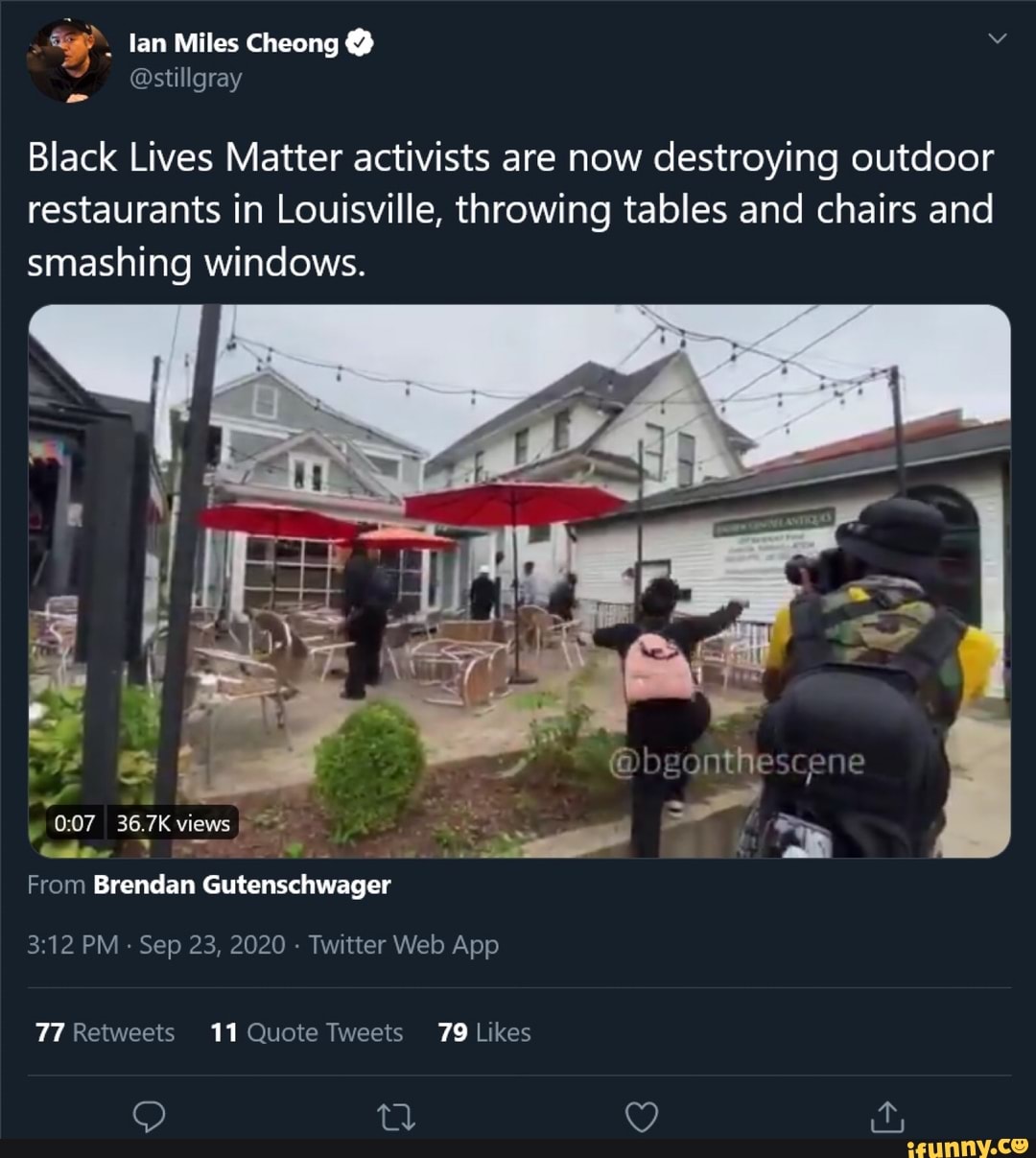The image depicts a screenshot of a tweet from Ian Miles Cheong (@stillgray), a verified Twitter user. The tweet is framed on a black background with white text and reads: "Black Lives Matter activists are now destroying outdoor restaurants in Louisville, throwing tables and chairs and smashing windows." Accompanying the tweet is a blurred, chaotic scene from a video clip. In the visual, there are clearly visible individuals seemingly attacking an outdoor restaurant setting. Tables and chairs are overturned, and red umbrellas are scattered amid the melee. String lights are hung across poles, adding to the ambiance of the outdoor space.

In the forefront, a person with a pink backpack appears to be aggressively charging towards the tables. Another individual, clad in a yellow shirt, black hat, and equipped with a backpack, is clearly photographing the incident, pointing his camera lens at the unfolding chaos. The video clip from which this scene is taken is 7 seconds long and has garnered 36.7K views. The timestamp on the video indicates it was filmed by Brendan Gutenschwager at 3:12 PM on September 23, 2020.